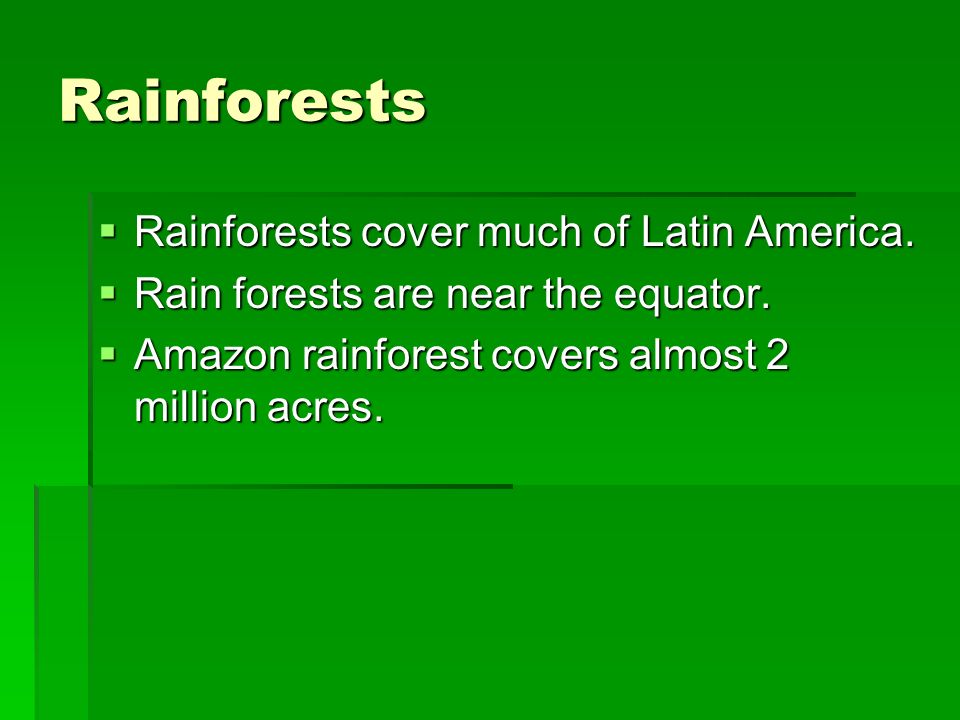The image is a detailed slide from a PowerPoint presentation, prominently featuring a dark to light green gradient background that evokes the lush greenery of a rainforest. The title "Rainforests" appears in a bold, rounded yellow font at the top left corner. Below the title, three bullet points are organized in a clean white font, each marked by a bright green square bullet. The bullet points convey informative facts: the first states "Rainforests cover much of Latin America," the second reads "Rainforests are near the equator," and the third highlights that the "Amazon Rainforest covers almost 2 million acres." The overall layout is simplistic and clean, with the lower third of the slide left blank, accentuating the gradient effect and keeping the focus on the text. There are no additional images or clip art, making the presentation straightforward and easy to read.